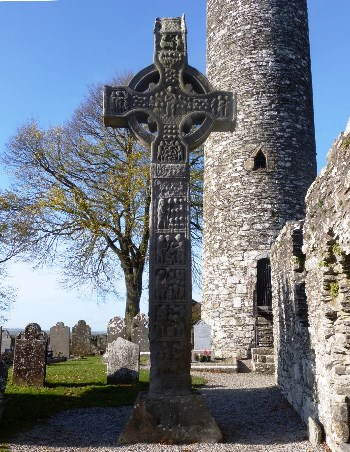This is a photograph taken at a cemetery, prominently featuring a very old, tall, and narrow stone cross with intricate 3D etchings and a circular feature around the intersection. The cross, of Gothic design, serves as the central focus of the image. To the right of the cross stands a large, brick, castle-like tower with a small pointed arch window halfway up, a doorway barred by shadowed stone steps, and a crumbling wall covered intermittently with moss. In front of this wall is another brick structure. The left side of the image displays several ancient, stone tombstones with traditional rounded tops, although the inscriptions on them are no longer legible due to age and dirt. In the background behind the cross, a sparsely leafed deciduous tree with slightly yellowed leaves and a half-bloomed canopy stands against a clear blue sky.